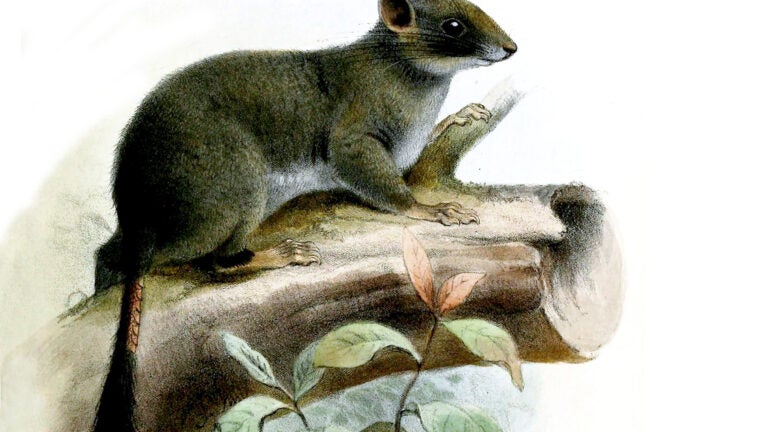This highly detailed color illustration, either painted or done with colored pencils, showcases a naturalist's sketch of an unidentified small mammal resembling a mix between a squirrel and a rat. The creature has a body and legs similar to a squirrel, with grayish fur on its back and legs that transitions to a white chest and underbelly. Its head is more akin to that of a mouse or rat, and it sports a unique tail that is partly bare like a rat's, but with a plume of fur at the end.

The animal is depicted sitting on the chopped-off end of a log or tree limb, facing right, with its tail trailing at the bottom left of the image. The log itself has a blunt, straight cut at the end, suggesting it was sawed off. Around the base of the log, there are herbaceous, shrubby plants with green leaves and reddish new growth adding a touch of color.

The artwork, inspired by an antique style of illustration found in natural history books, focuses on the animal and its immediate surroundings against a white backdrop, emphasizing its features and habitat details.